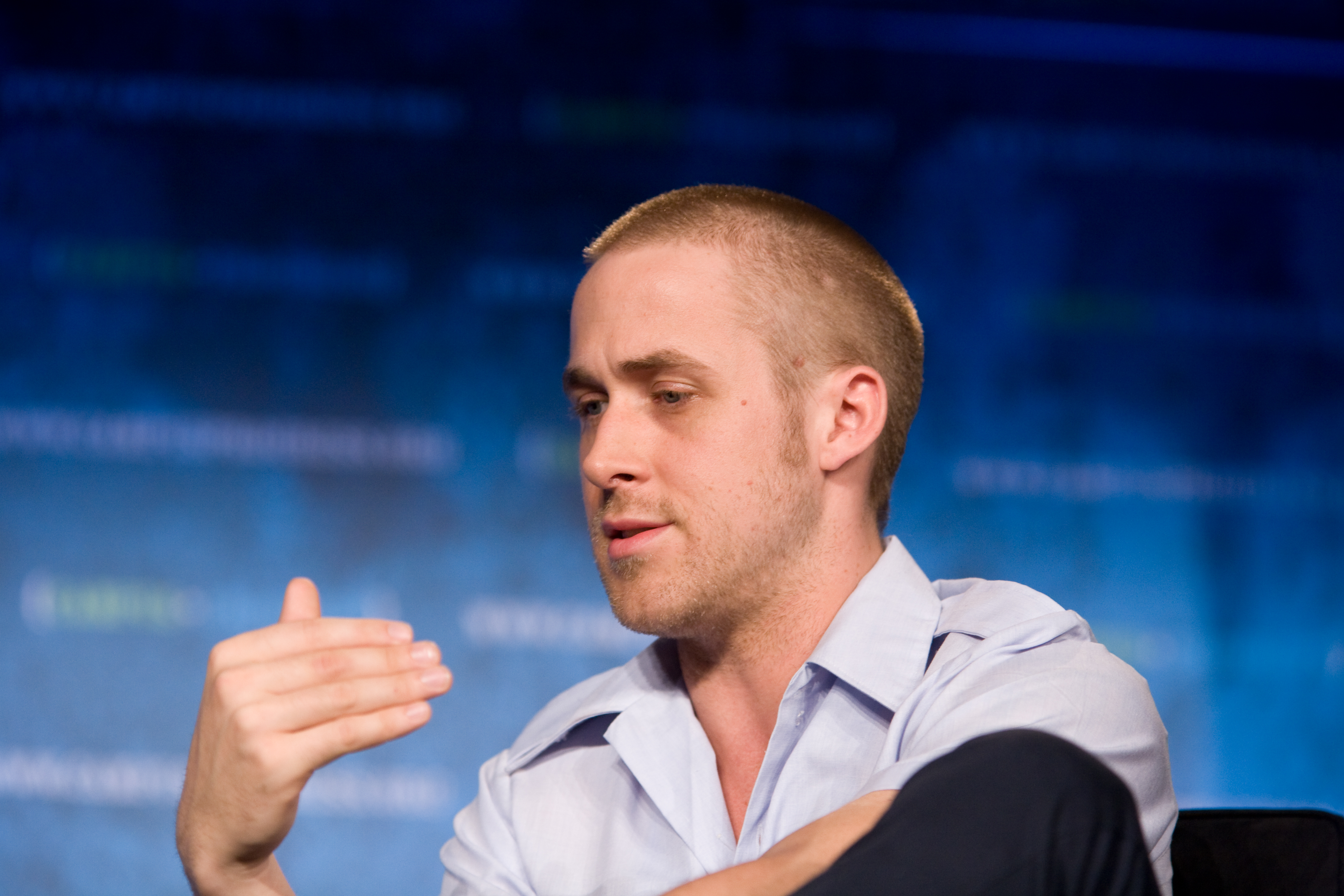This detailed, colorful portrait features a man resembling a famous actor, albeit not Ryan Gosling, estimated to be around 40 years old. Captured in a close-up shot cropped at the shoulders, he dons a short-sleeved, light blue shirt and black pants. His light brown hair is closely shaved, coupled with faint sideburns, a light beard, and a light goatee. The man is in mid-conversation, looking to his left with a raised hand gesture, possibly speaking at a conference or an interview. He is seated on a black chair, with only the top of his knee visible. The backdrop is a blurred, navy blue screen with white weathering or possibly a PowerPoint slide, lending an undefined and indistinct quality to the scene behind him. The photograph is square, approximately six by six inches, focused on his face and expressive gesture, devoid of any discernible objects other than the chair.